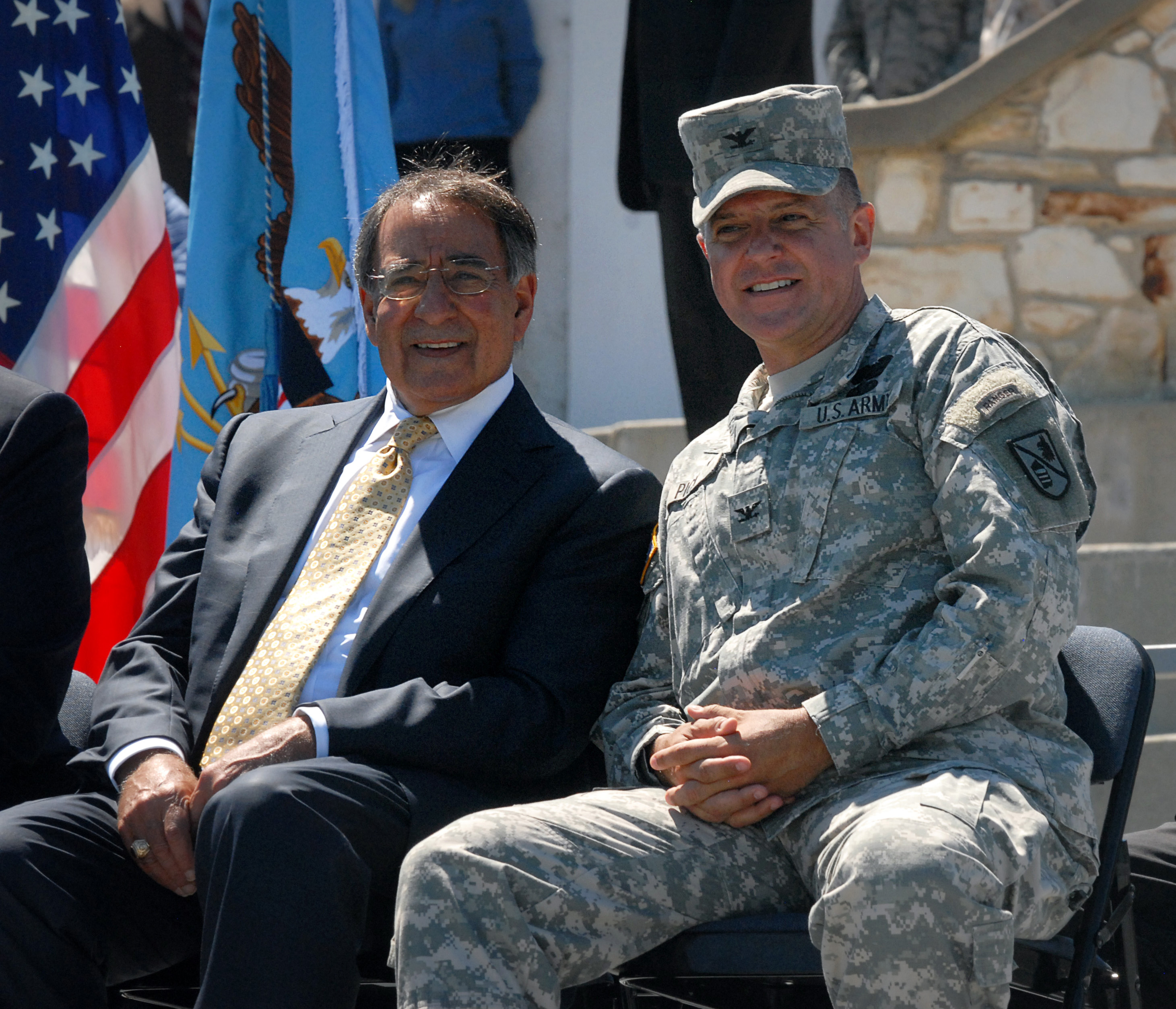In this detailed image, two men are seated in black folding chairs, side by side, both smiling. The first man, a soldier, is dressed in grayish-green U.S. Army fatigues adorned with various badges on one arm and a crest on the other. His uniform also prominently displays "U.S. Army" on his chest. He wears a matching hat and has his hands resting in his lap. Next to him sits an older gentleman, perhaps in his late 60s or 70s, dressed in a black suit with a white collared shirt, a yellow and blue tie, glasses, and a notable ring on his finger. Behind them, the backdrop includes an American flag along with a light blue military flag featuring a bald eagle with brown wings, a white head, and a gold beak, and holding arrows. There are also other people standing in the background, adding depth to the scene.